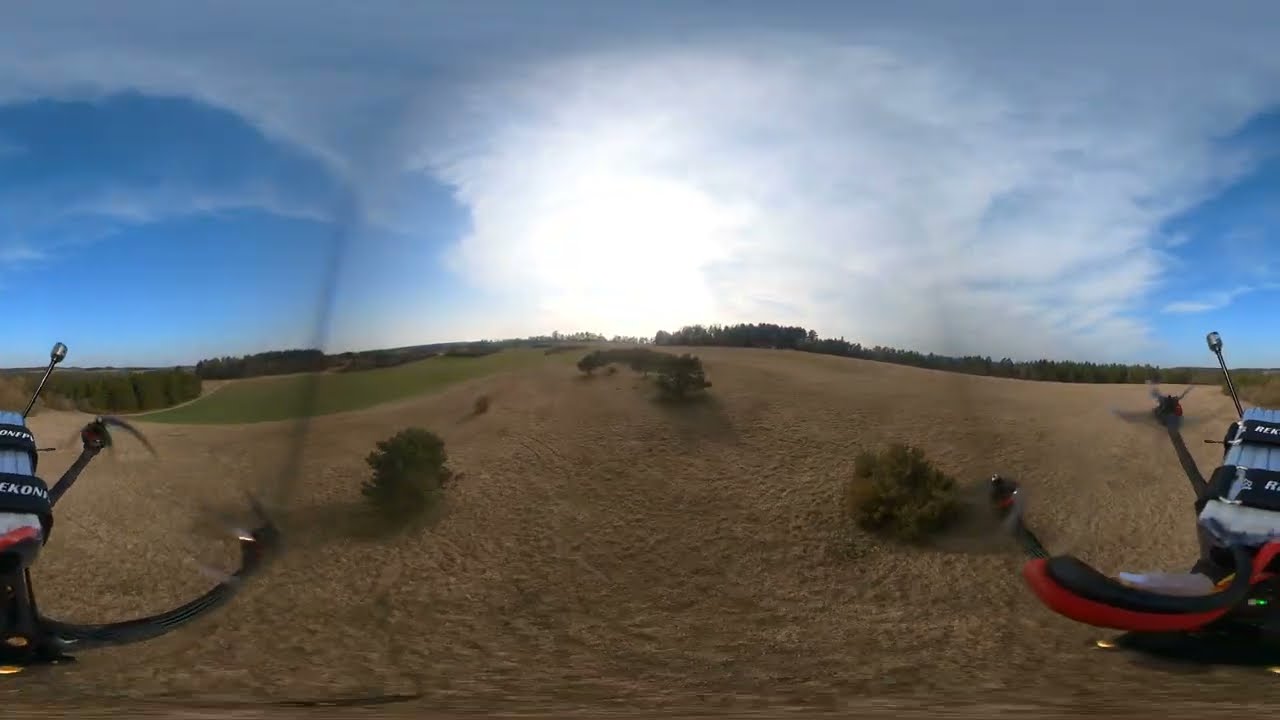This is a horizontally aligned rectangular picture taken outdoors, possibly from a drone or through a motorcycle's front shield, given the visibility of partial devices on the left and right sides of the image. These devices, including a black gear on the left and a red and black brake lever on the right, occupy roughly a quarter of the image combined. The center appears blurry, indicative of the photo possibly being taken through a window-like surface. The scenery features an open field with predominantly brown or yellowing grass, suggestive of fall or early winter. There are a few small green bushes in the foreground and a patch of green grass on the left side of the frame. Further in the distance, a line of trees forms the midground. Above, the sky features a mix of blue and cloud formations, with the sun shining brightly through the clouds, casting a bright white area in the middle. The sky transitions to a more blanket-like gray at the very top, while the horizon shows hints that the sun is either rising or setting.